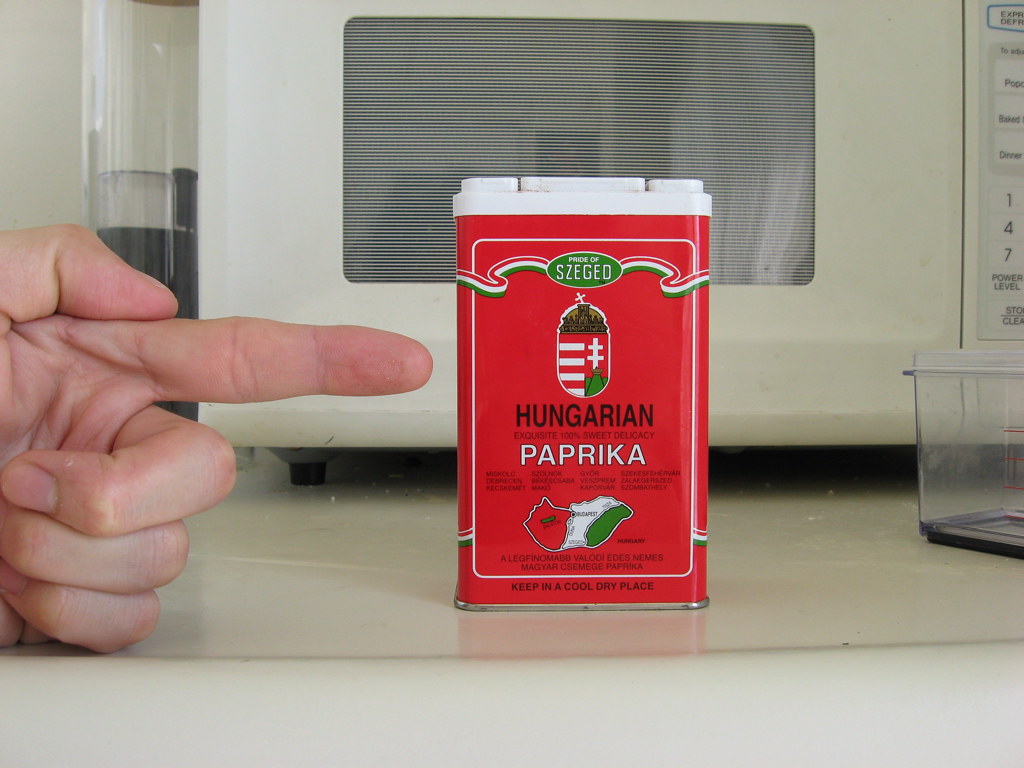The image features a close-up view of a metal container of Hungarian paprika, prominently branded as "SZEGED." The container is red with a white plastic top that includes multiple lids suited for both spoon dipping and direct shaking. An individual's finger is visibly pointing at the container, with the thumb resting on the pointing finger and the other fingers curled back. The text "Keep in a cool, dry place" and "Product of Hungary" are printed on the container, highlighting its origin and storage instructions.

In the background, a small vintage microwave oven adds to the scene's ambiance, hinting at an older kitchen setting. To the right of the paprika container sits a plastic storage container, while on the left, there is a vial that could either be a part of a coffee maker or an accessory related to its use. The paprika container is placed on a flat surface, surrounded by these everyday kitchen items, emphasizing its role in a typical culinary environment.